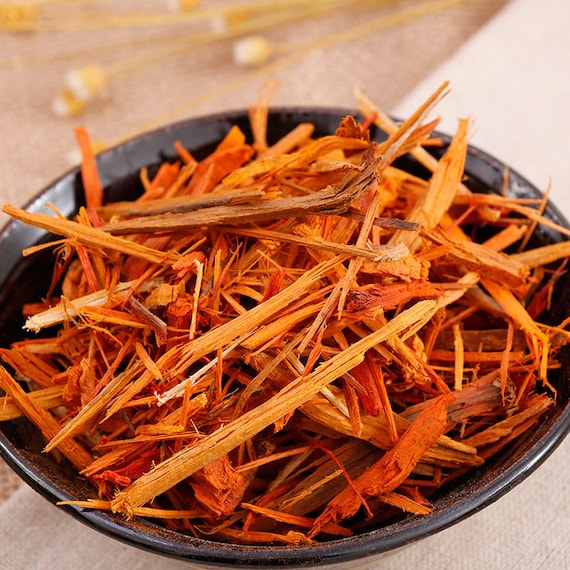In this vividly colored image, the focal point is a black pottery bowl, slightly shiny with minor imperfections, filled with assorted shards and slender sticks of wood. The wood pieces, piled together, range in shades from light to dark orange, reminiscent of redwood or cedar bark, and some resembling the texture of sweet potato chips. The bowl is situated on a white, smooth-looking surface. The background, slightly blurred, features golden reed-like objects with white, puffy cotton ball tips, set against a beige backdrop. The overall composition highlights the striking contrast between the bright orange wood and the dark bowl, creating a visually compelling and artistic arrangement.